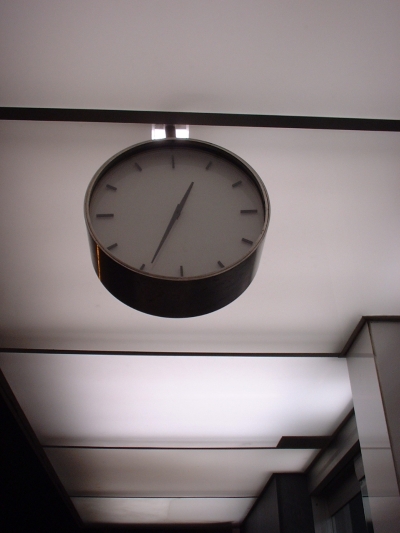In this image, a round clock is mounted on a panel or the ceiling, positioned above a doorway or at the entrance of a hallway. The clock features a metallic, metal-like border and is covered with a translucent material, likely plastic or glass. Instead of conventional numerals, the clock face is marked by 12 small slashes, arranged clockwise. The clock has an hour hand that is shorter than the long, slender minute hand. The time displayed is approximately 12:34. The ceiling, which is brightly illuminated, appears to be lit by fluorescent lights. As we are looking upward, the view of the hallway is obscured, focusing our attention primarily on the clock and the brightly lit, white ceiling.